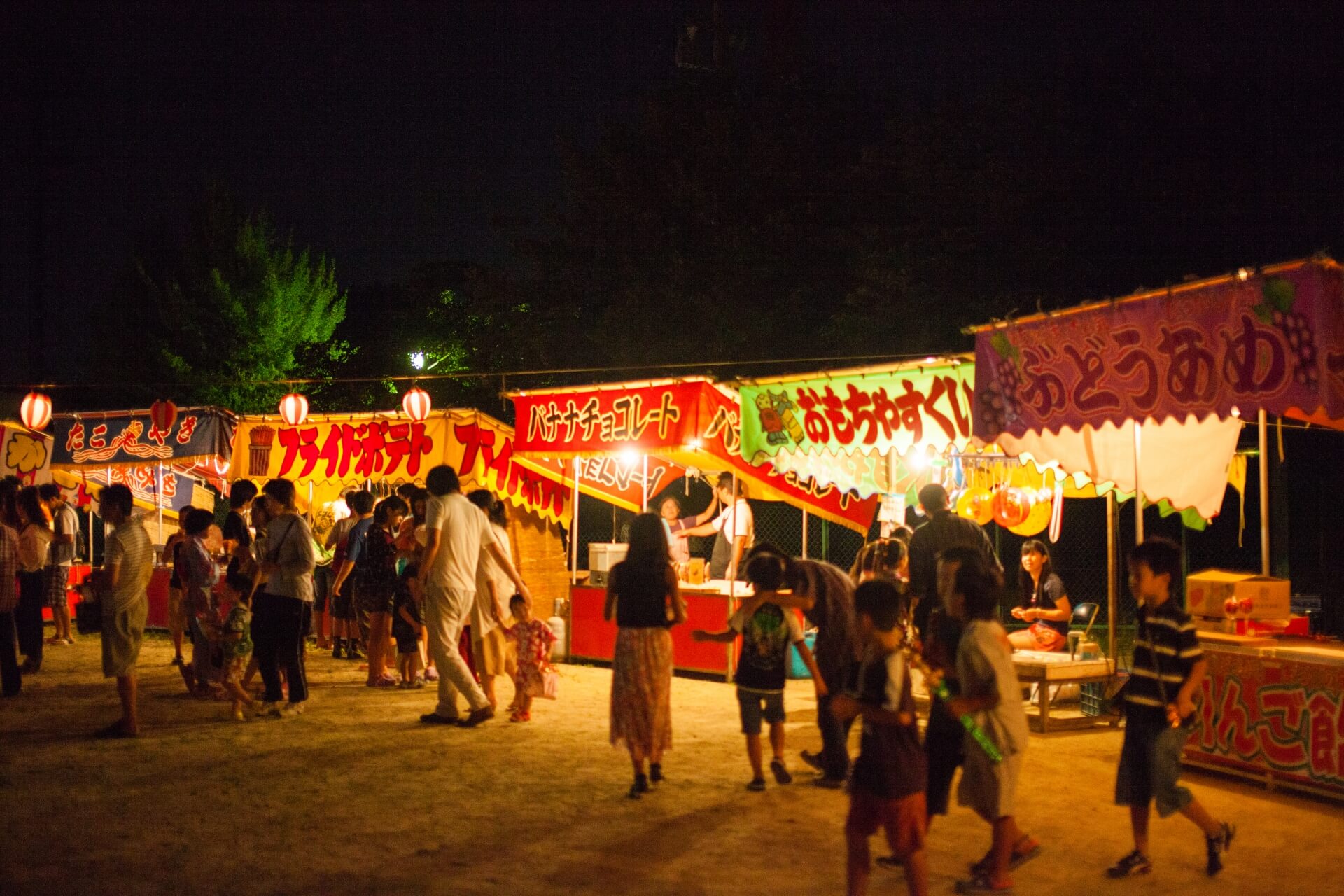This nighttime image captures a bustling festival, most likely located in the Far East due to the presence of Asian lettering on various colorful canopies and awnings. The sky is jet black, contrasting with the vibrant activity below. Strings of circular hanging lights traverse the scene, illuminating the gathering and adding a festive atmosphere.

Multiple food vendors line the space, each under brightly colored banners: a prominent orange banner with brown symbols, a red banner against a white background, another with black letters on red, a yellow one with red letters, and a dark blue one with light yellow lettering. Each stall is attended by numerous patrons, hinting at a wide array of culinary offerings.

In the lower right, a young boy in a striped black and gold t-shirt and shorts stands next to two other children dressed similarly in shorts and t-shirts. Nearby, another group of children holds light-up swords, indicating the presence of playful, family-friendly activities. In the center, a woman in a long dress and black blouse approaches one of the vendors, while a man in an apron tends to a cooking pot, reinforcing the food-centric nature of the event.

On the left, green trees and a street light slightly illuminate the area, which is populated with families and individuals of all ages walking on what appears to be a dirt ground. The festival atmosphere is lively and inviting, clearly depicted by the movement and interactions of the crowd.